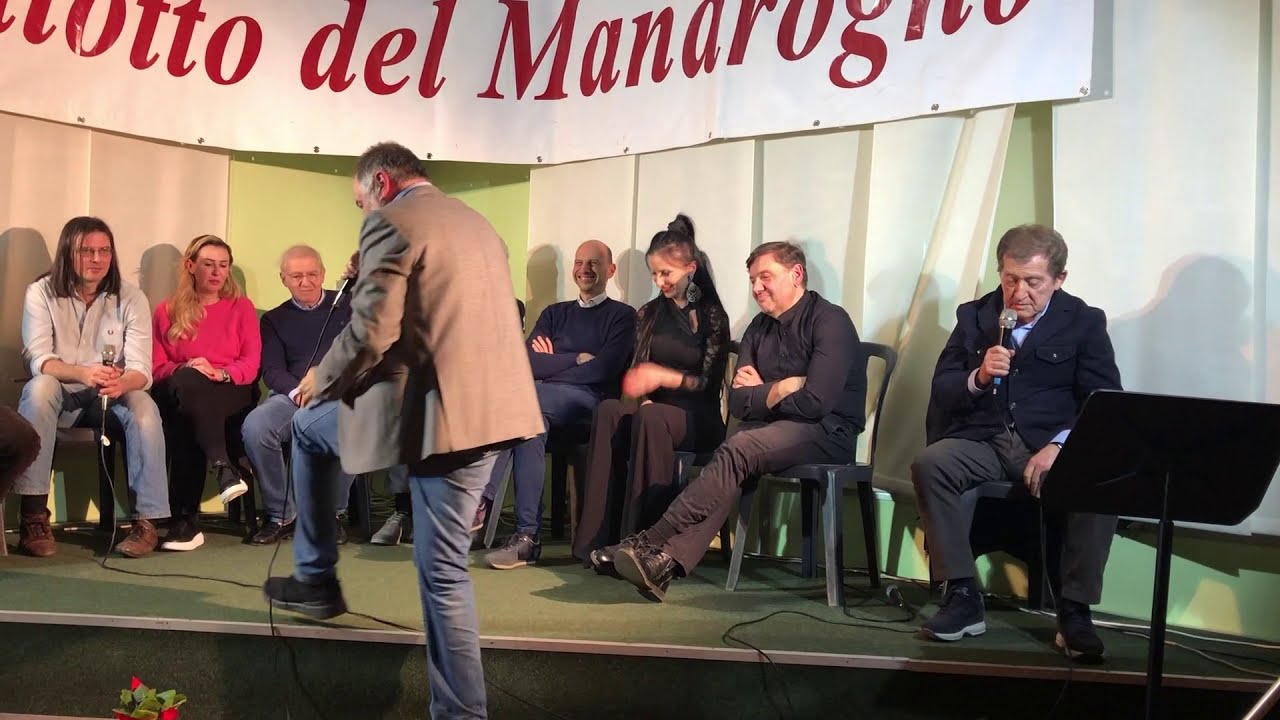The image is a horizontally aligned rectangular photograph capturing an event or ceremony, possibly a conference or church service. On the stage, which has a green floor, ten people are seated in chairs, a mix of men and women ranging from middle-aged to elderly. Behind them is a backdrop made of white sheets of paper partially obscuring a green wall. Above the seated individuals hangs a large white banner with red lettering, partially cut off, reading something like "Motto Dell" and "Monoragno," suggesting text in Italian or Spanish. A man with a brown sport jacket and blue jeans is stepping onto the stage with a microphone in hand. On the far left, another man holds a microphone, while on the far right, yet another man, dressed in a dark coat and gray slacks or jeans, is speaking into his microphone. Other participants are smiling and observing the man stepping up.